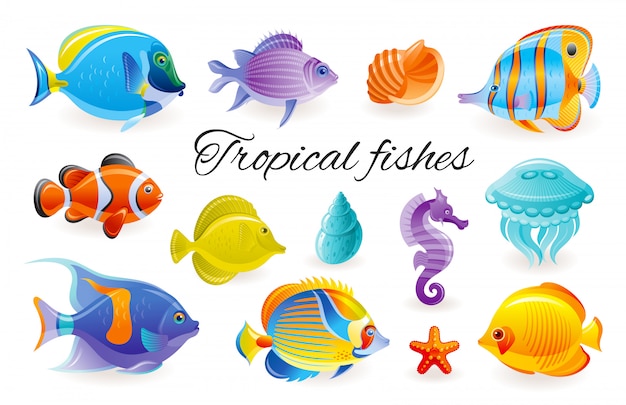The image features a stark white background with no visible borders, emphasizing a clean and minimalistic design. At the center of the image, in a swirly, cursive black font, the phrase "tropical fishes" is prominently displayed. Surrounding this central text is a grid of computer-generated, cartoonish sea creatures arranged in landscape orientation. The grid consists of four rows with varying numbers of creatures in each row: the top row has three fish and one shell, the middle has a combination of five creatures including two fish, a shell, a purple seahorse, and a teal jellyfish, while the bottom row showcases three fish and a small starfish.

The sea creatures are vividly colored, featuring hues such as bright orange, yellow, teal, purple, blue, and green. Specifically, the lineup includes a typical clownfish reminiscent of Nemo, a yellow angelfish, an orange-yellow fish, and a starfish, amongst other assorted tropical species. The shells add an additional splash of color with their teal and orange shades. This whimsical and vibrant image, with its cartoon-like aesthetic, could easily find a place in a child's room as an engaging and educational piece of decor.